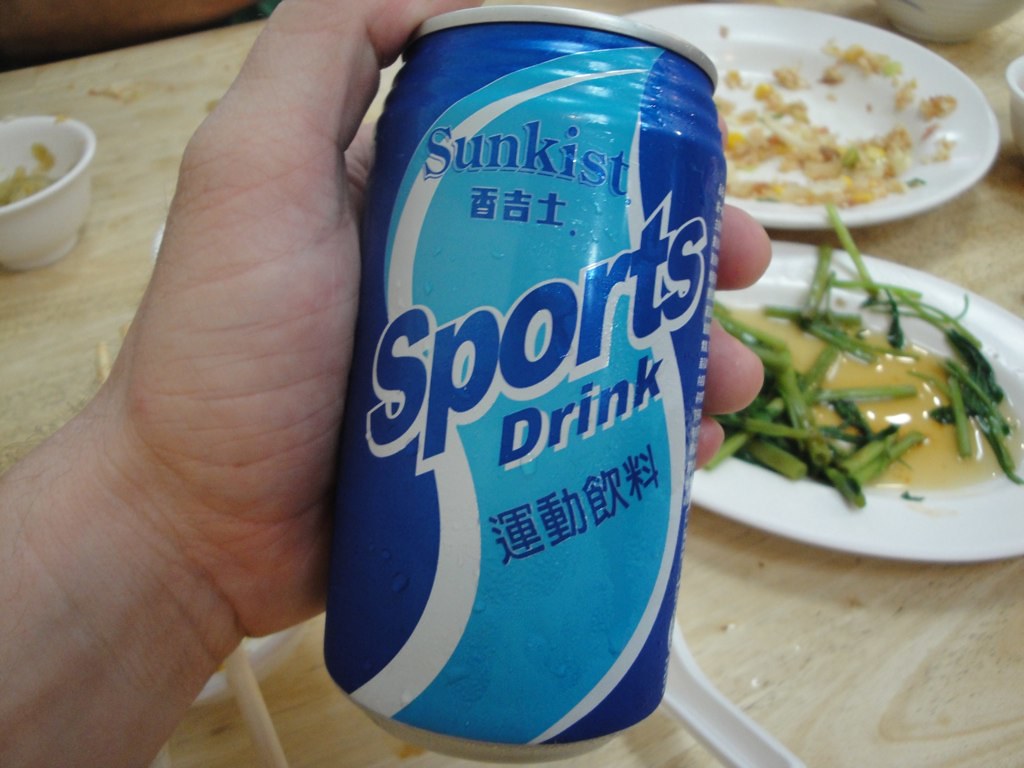The image features a Sunkist Sports Drink can prominently held up close to the camera by a light-skinned person's left hand. The can is primarily blue with wavy white and light blue sections, and it bears the text "SUNKISSED SPORTS DRINK" along with some Japanese or Chinese characters underneath. The person's thumb is positioned at the top of the can, while their remaining fingers grip its main section. The background showcases a light wooden surface adorned with various dishes. On the right, there's a partially finished plate of fried rice and another plate containing green vegetables, possibly scallions, in some sort of broth. Additionally, in the upper left corner, there is a small ramekin with an unidentified green and yellow food or sauce. The overall color palette of the scene includes shades of blue, white, green, yellow, and light beige.